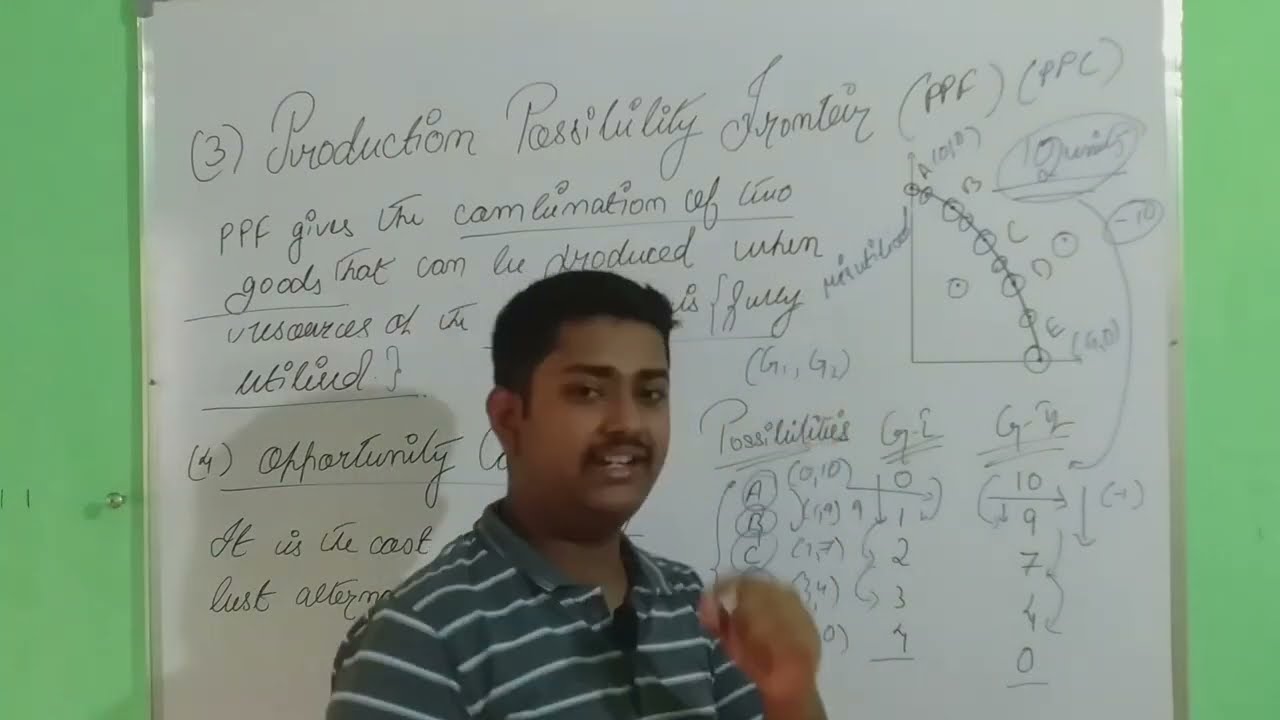The image showcases a photorealistic depiction of a South Asian man standing in front of a large whiteboard, affixed to a bright green wall on both ends. He has short, dark black hair and a distinctive, neatly trimmed black mustache that is squared off. The man is dressed in a blue collared shirt with fine white stripes. He is gesturing animatedly with his right hand, which appears slightly blurred due to motion, suggesting he is in the midst of explaining or emphasizing a point.

The whiteboard behind him is densely covered in predominantly cursive-like black writing. On the left side of the board, most of the content consists of words, featuring terms like "Production Possibility Frontier" and "PPF gives a combination of two goods that are produced when resources." On the right side of the board, there are numerical data and a chart graph, likely associated with the formulaic expression he is teaching. Although some parts of the text are obscured by his presence, it is evident that he is engaged in providing a detailed explanation, possibly relating to economic or business formulas. The bright green wall on either side of the whiteboard further enhances the vividness of the scene.